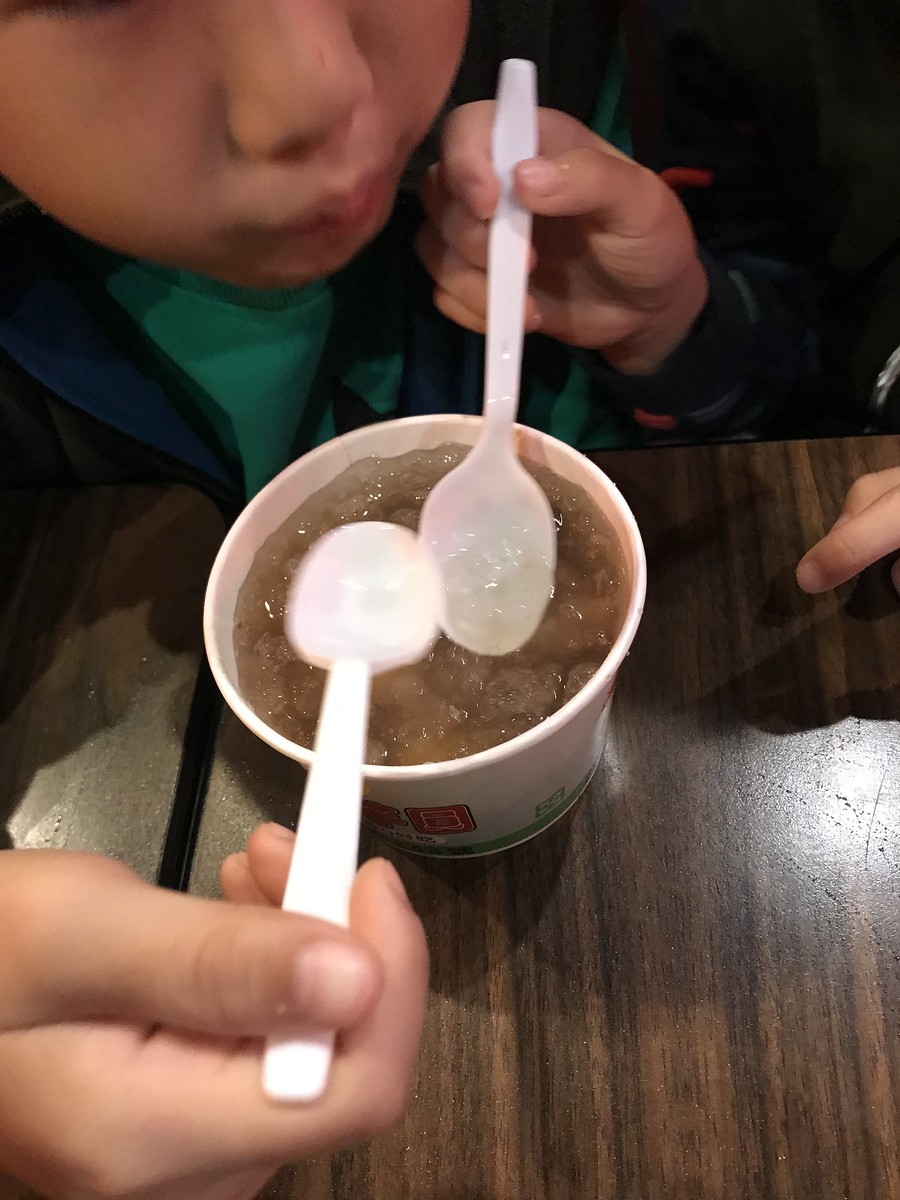In this photograph taken in a dark room, the background is not visible, but the focus is on a wooden tabletop. At the table sits a young boy, likely of Asian heritage, dressed in a green shirt and a blue jacket. He is smiling, holding a white plastic spoon. Another white plastic spoon is held by a hand entering from the edge of the image, and both spoons are dipping into a white paper cup containing a light brown liquid with ice, possibly a type of soda. Additionally, a third hand, with its fingertips just visible on the right side of the image, does not hold anything. The scene captures a moment of shared activity and enjoyment, with the boy's smiling expression suggesting a happy, content moment.